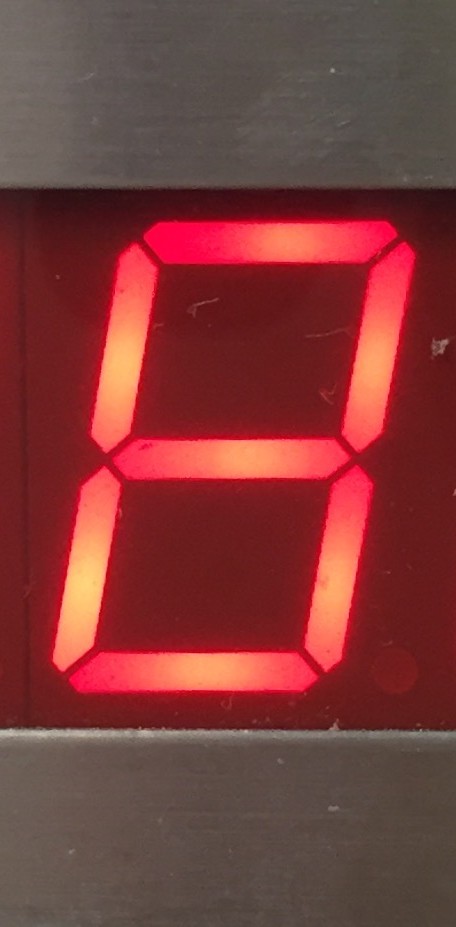The image features a detailed close-up of the number 8, displayed on a digital screen. This digit appears slightly leaning to the right and is composed of seven illuminated bars—three horizontal and four vertical. These bars are illuminated in varying intensities of orange and yellowish shades, with some parts brighter, particularly along the sides. The background of the image is a dark red color, enhancing the contrast with the illuminated 8. The top and bottom edges of the photo feature black and gray-silver metal, possibly the casing of the digital screen. Furthermore, there are small fibers of dust or hair visible against the black sections and within the spaces of the 8, adding a touch of realism to the digital display.